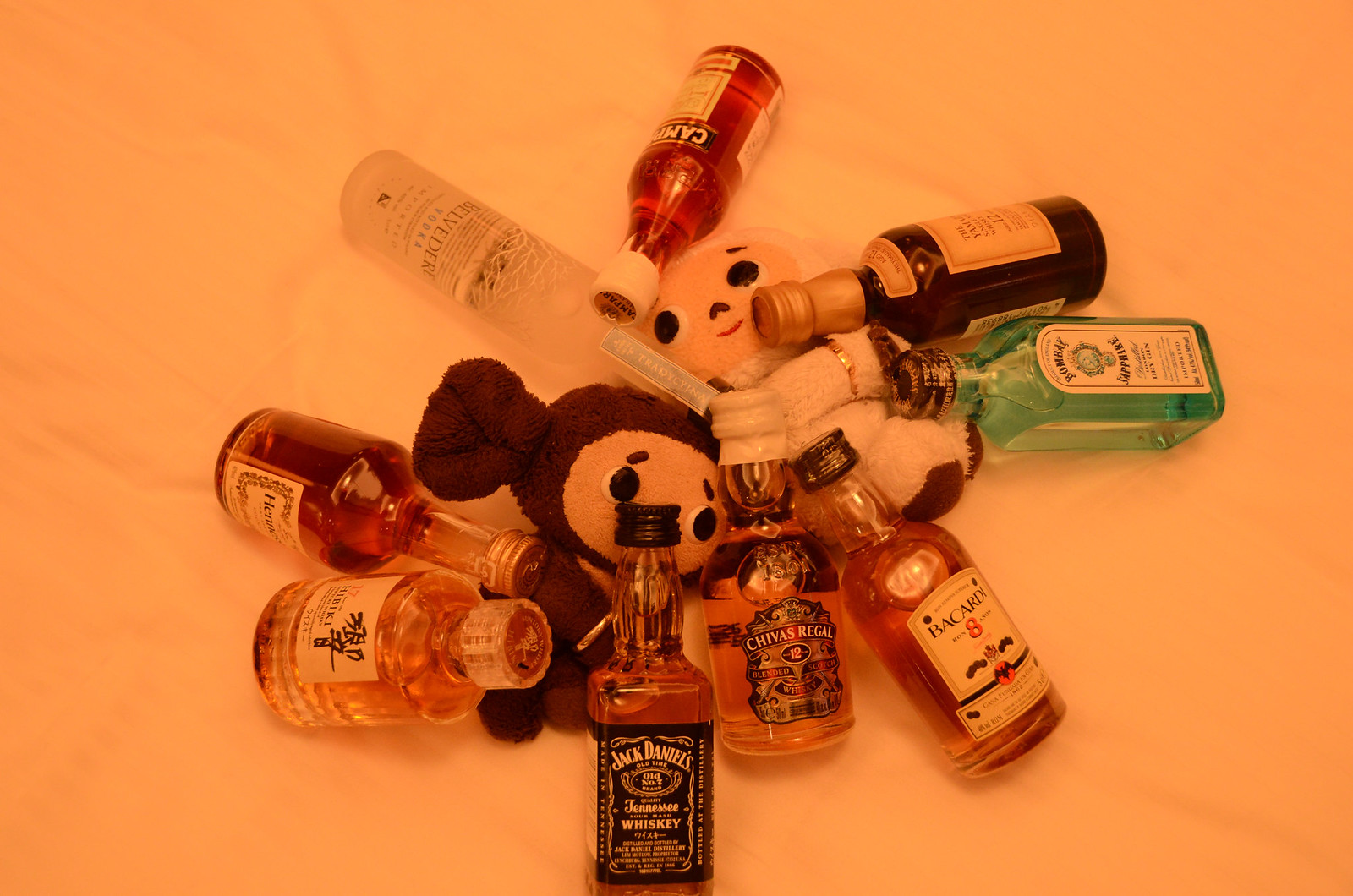This edgy photograph, reminiscent of an early 20s aesthetic, captures a chaotic yet charming scene from a probable domestic setting with a peachy, pink-orange backdrop. 

Taken from an overhead perspective, the image features two stuffed animals partially obscured by an assortment of miniature liquor bottles. The first stuffed animal, possibly a brown mouse, has large oval-shaped ears, a pale tan face, and expressive large eyes with arched eyebrows that convey a concerned look. The second stuffed animal, primarily white or off-white, has its head obscured, but visible features include brown circles on its feet and a red smiling mouth with eyes looking upwards and to the left.

Surrounding these dolls are an array of miniature alcohol bottles, including recognizable brands such as Jack Daniel's Tennessee Whiskey, Chivas Regal, Bacardi, Bombay Sapphire, Campari, Belvedere Vodka, and Hennessy. These bottles vary in color, predominantly amber, brown, or dark yellow, with a striking blue bottle, perhaps Bombay Sapphire, adding a vibrant contrast to the palette. Some labels are written in Japanese or are turned at such angles that they are unreadable. The combined details of the plush dolls and the carefully arranged miniature bottles create a visually captivating and detailed portrayal of a whimsical yet edgy vignette.